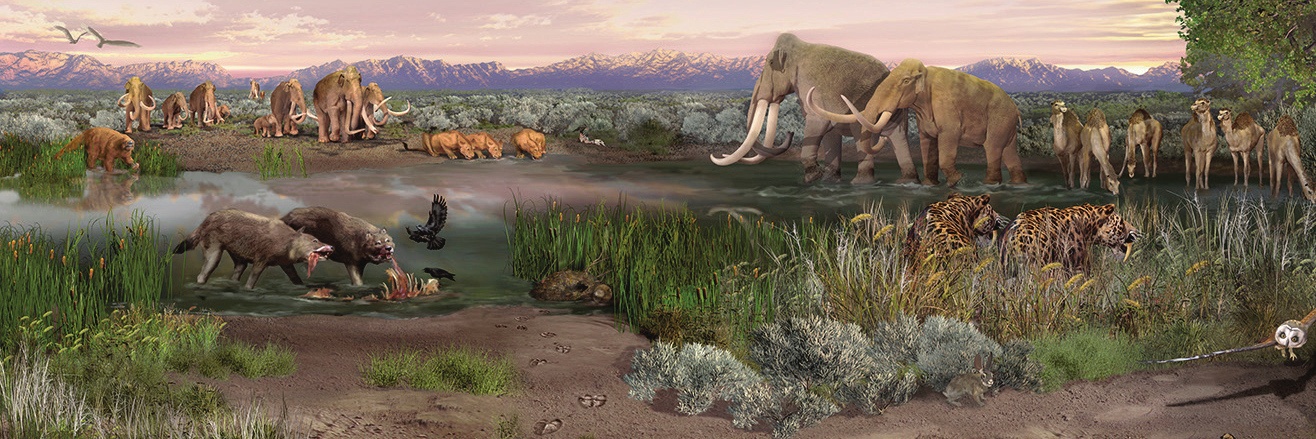The image depicts a richly detailed, prehistoric scene that appears painted or digitally rendered. In the foreground, brown dirt transitions into green shrubs and light blue water, with a small jackrabbit near the front. To the left, wolves are seen consuming a carcass partially submerged in water, backed by saber-toothed tigers drinking from a lake. An imposing giant sloth is also by the lake, while a pack of woolly mammoths march towards the water. On the right, further in the water, additional woolly mammoths are found beside some camel-like creatures. Close to the riverbank, long-tusked leopards survey their surroundings. The scene also includes a low-flying owl and birds scattered across the purple sky, painting a vibrant picture of a primeval landscape. The midsection of the image blends grassy patches with dirt, featuring vegetation such as tall grass and little bushes, resembling a grassland. In the distant background, purple mountains rise under a matching sky, adding depth to this ancient panorama.